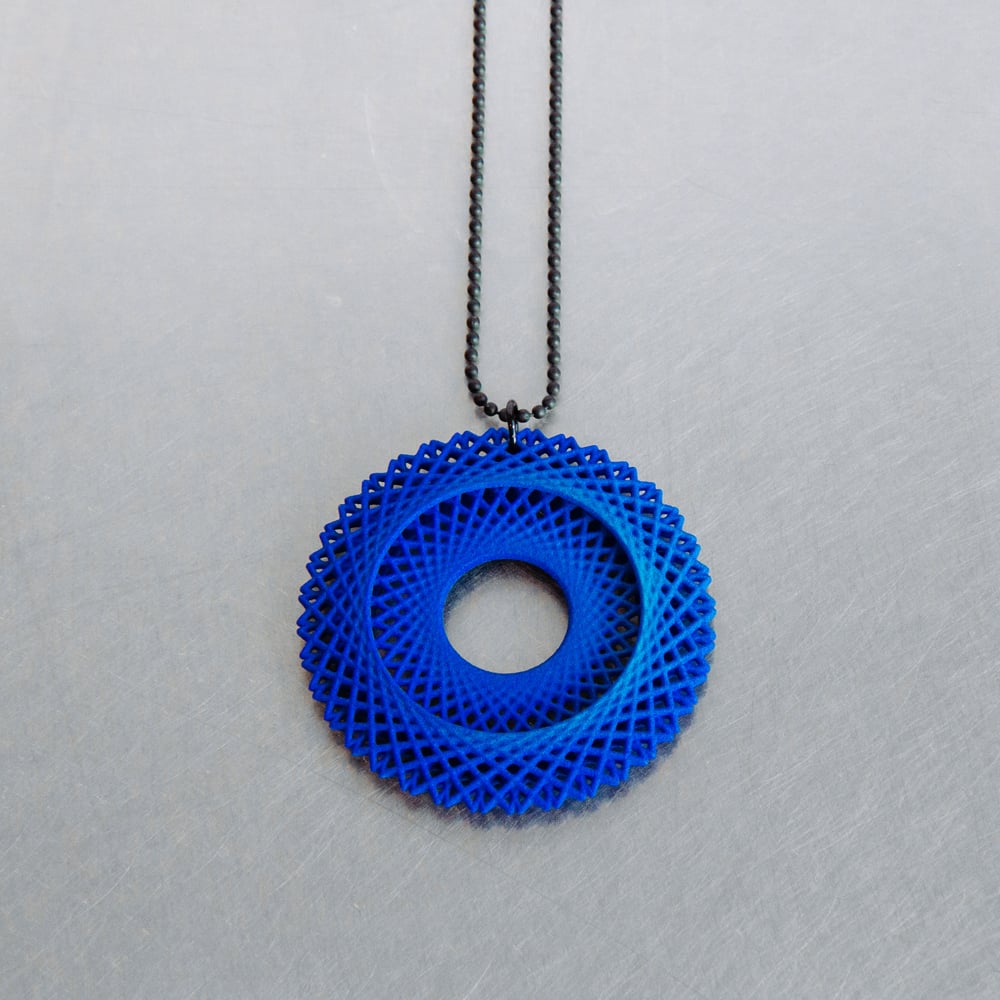The image features a black beaded necklace with a fisheye clasp, artfully draped on a light gray background streaked with white. The necklace centers around an intriguing blue, spirograph-inspired medallion. This medallion consists of two concentric circular designs, intricately detailed with lines and patterns that intersect to form a large netted outer ring and a clear inner ring with a hole in its center. The black necklace extends from the top of the image and loops back, seamlessly blending with the monochromatic background.